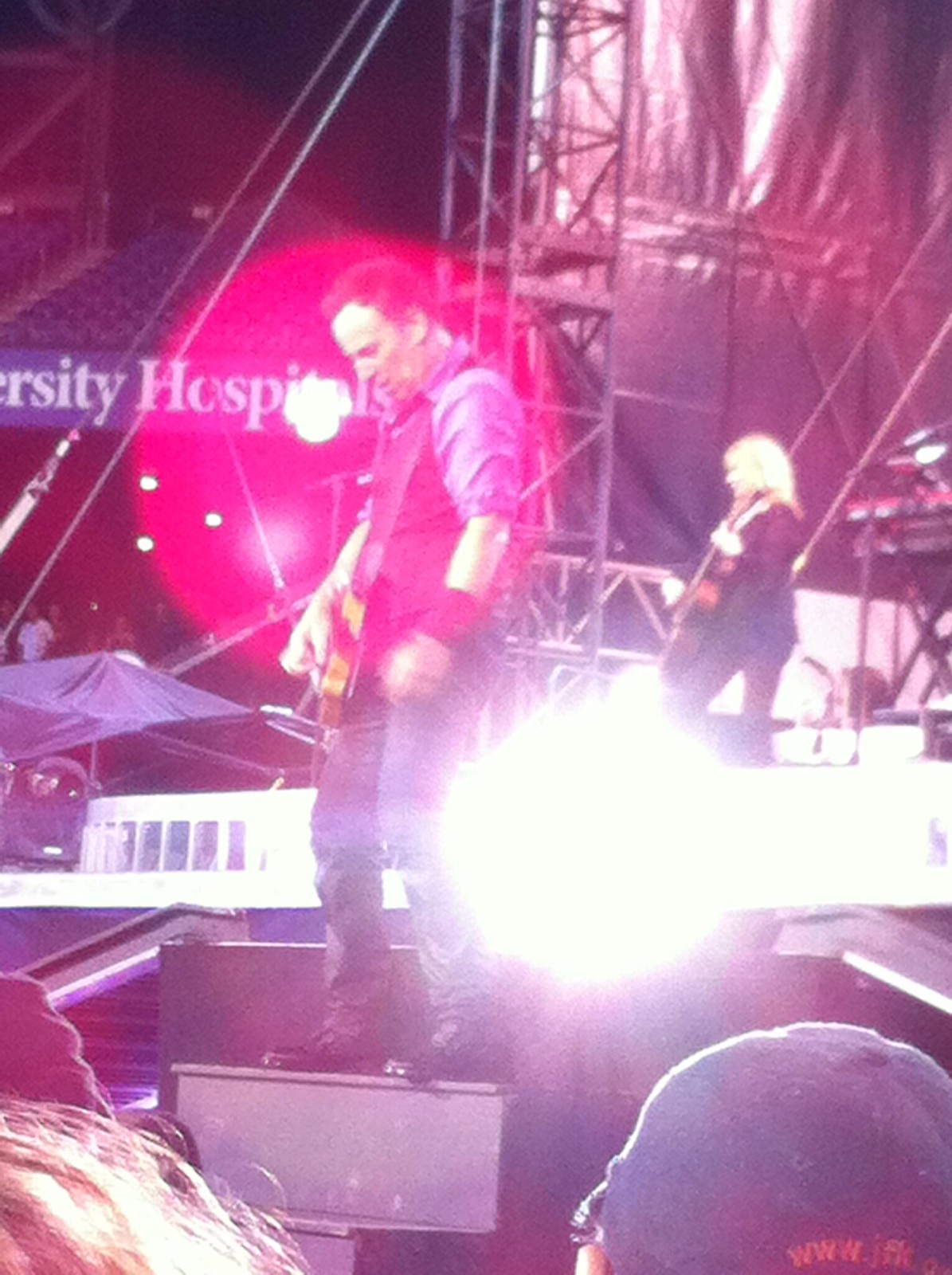The image captures a live concert scene taken from the perspective of the crowd, close to the front of the stage. The foreground reveals the tops of two heads, one wearing a baseball cap and the other with visible long hair. On the stage, a male guitarist, possibly resembling Bruce Springsteen, is the focal point. He is dressed in a rolled-up shirt with a vest, jeans, boots, and a dark wristband. He holds an electric guitar and looks downward, immersed in his performance. Behind him, bright lighting creates a burst of pink light, adding a dramatic effect to the scene.

Also on the stage, a female guitarist with blonde hair, clad in a long-sleeve black shirt, holds an acoustic guitar. She is positioned towards the back and looks to the side, partially obscured by stage equipment and a large black tarp. The overall setup includes rigging, towers, and additional lighting, with crew members stationed off to the side.

A prominent banner reading "University Hospital" hangs above the stage, partially obscured but discernible. The audience is faintly visible in the middle background, with some empty seats pointed out towards the upper left. The vibrant atmosphere suggests a live performance in progress, capturing the energy and memory of the moment.